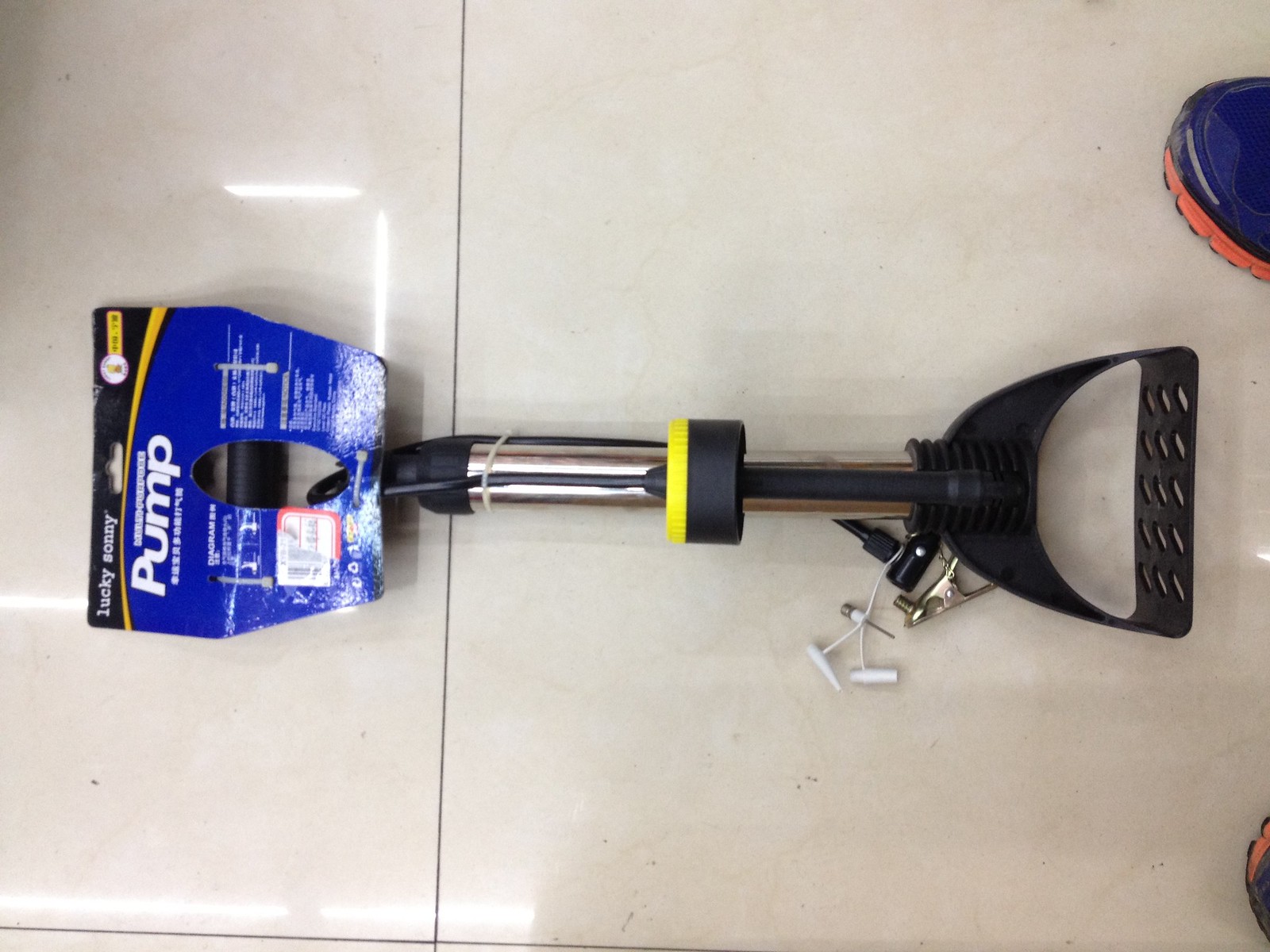The image depicts a bike pump laying on a glossy white surface, possibly a desk or tile floor, reflecting fluorescent lighting. The pump's packaging, located at the top left, features a black vertical banner with unreadable white text above a blue section that prominently displays "Lucky Sunny" and "PUMP" in large white letters, alongside some Chinese characters. The pump itself has a metallic cylindrical body with a black and yellow ring encircling its middle. The handle at one end of the pump is black plastic, and at the other end, it terminates in a component that resembles an ice scraper with a hole in the center and small cutouts on the edge. Scattered next to the pump are some screws and bolts. In the background, a partial glimpse of a person wearing a blue and red shoe is visible.